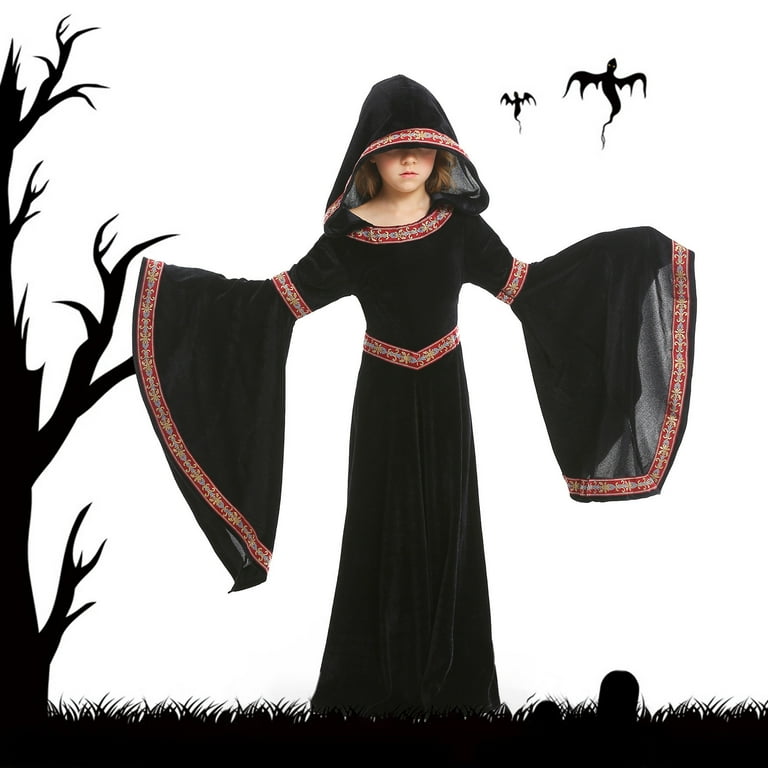In this Halloween-themed photo, a young girl, possibly between the ages of 7 to 11, models an elaborate costume that blends elements of a witch and a medieval princess. She wears a long, black dress made of velvet or velour, adorned with intricate red trim that is detailed with a white and gold pattern. The dress features a large hood that envelopes most of her face, leaving only her nose and mouth visible, reminiscent of Morticia from "The Addams Family." Her large sleeves flair dramatically, extending well past her hands as she holds her arms spread wide.

The background is predominantly white and appears to be a drawing with dark, eerie elements. To the left, a menacing, leafless black tree stretches its barren branches. Below it, black grass spreads across the bottom of the image. On the right, a small black tombstone stands ominously. Above the girl to the right, two silhouetted bat-like ghouls with wings outstretched add to the spooky atmosphere. The depiction of these ghouls, along with the overall design elements, give the impression of a haunted scene, framing the girl as an enchanting yet eerie figure.